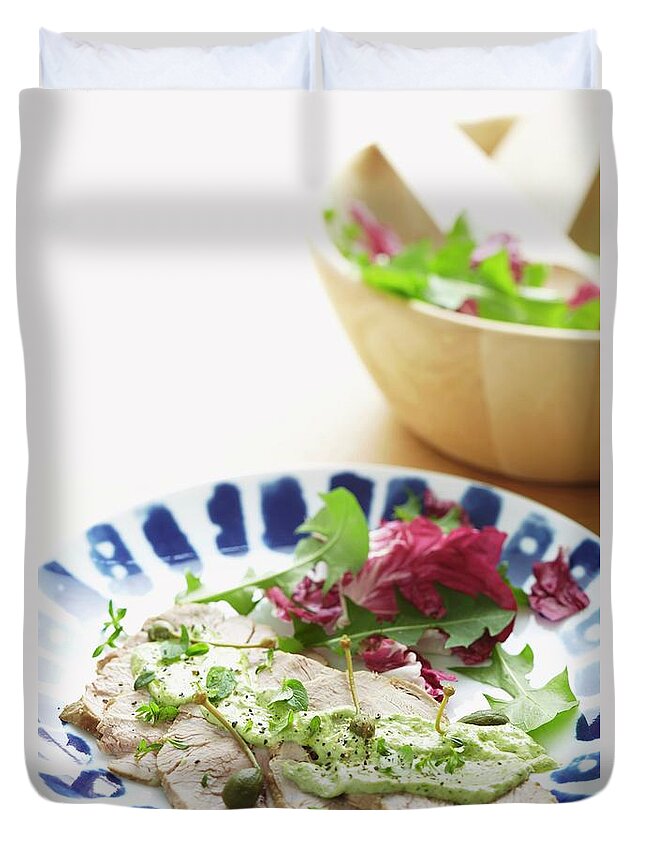The image features a neatly made bed with a white bedspread and matching white satin pillows at the head. Captured from a top-down view, the bed is adorned with an intricate illustration of a meal. The illustration on the white bed sheet depicts a white plate with blue edges, artfully arranged with sliced chicken bathed in a thick, flavorful green sauce that resembles a pea mash. The dish is garnished with vibrant green leaves and sprinkled with magenta and green salad leaves, adding a burst of color. Adjacent to the plate, on the right side, sits a brown and white wooden bowl containing a mix of red and green salad leaves, similar to those on the plate. The detailed depiction of food creates a visually appealing and thematic setting on the bed's white background.